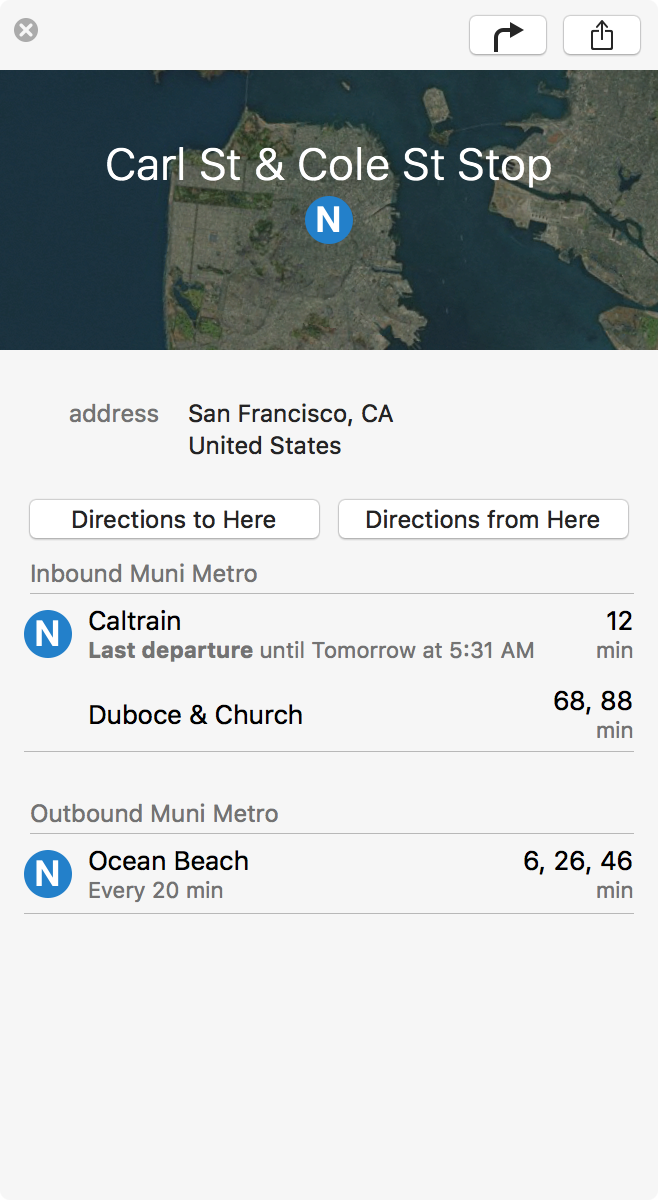The image features a user interface with a light gray background and various elements. In the top left corner, there is a gray 'X' icon. Alongside it are two buttons: one with a black arrow indicating a right turn, and another with a share icon, represented by a square with an upward arrow.

Central to the image is a map indication of the Carl and Cole Street stop for the N train. This stop is marked by a night-blue circle with white text reading "N." Below the circle, an address is given in gray text: "San Francisco, CA, United States," followed by specific address details in black text.

Two action buttons are positioned beneath the address: "Directions to here" and "Directions from here," both with black text on a light background and featuring rounded rectangle shapes.

Further down, information on inbound and outbound Muni Metro services is presented. For inbound services, there is a gray text label "Inbound Muni Metro" followed by the N train icon, indicating the last Caltrain departure being at 5:31 AM. This section lists specific timing details for Dubachi and Church at 12, 68, and 88 minutes.

A gray horizontal line separates inbound from outbound information. Under the "Outbound Muni Metro" section, grey text introduces the N train headed toward Ocean Beach, running every 20 minutes. To the far right, the times 6, 26, and 46 minutes are specified under another gray horizontal line.